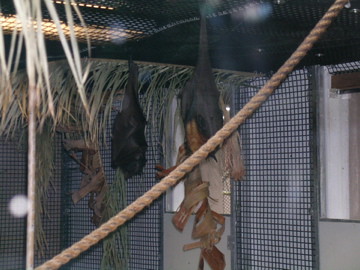The photograph depicts an indoor scene dominated by a net mesh structure. The mesh fabric extends across the ceiling and the sides of the room, creating a layered, intricate pattern. Hanging from this structure, there are strands of long green and white grass, interspersed with brown leaf bits, which add a natural, textured element to the space. A long, brown rope stretches diagonally across the front of the image from one corner to the other. Above the mesh canopy, a fluorescent light casts a white glow into the room, highlighting the mesh details and the suspended grass. The background features a dividing curtain that is partially open, offering a glimpse into an adjoining room with checkered blue walls. A mirror is visible on the wall of the outer room, reflecting parts of the scene and adding depth to the composition.